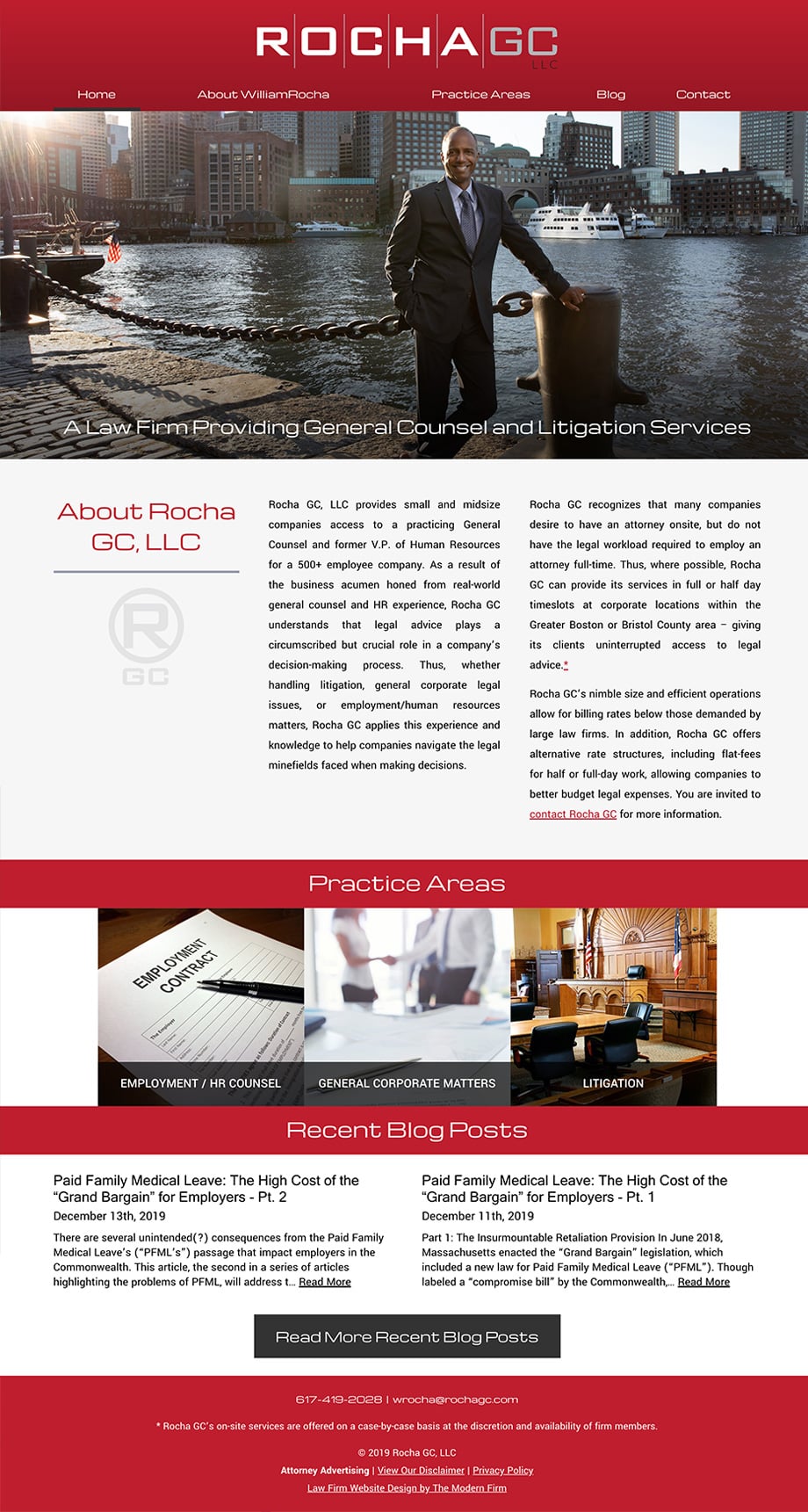This is a detailed caption for the provided image:

---

The screenshot captures a web page with a structured and professional layout. At the very top of the page, there's a bright red banner displaying the website's branding, featuring the logo "Rocha G.C. LLC" in large white letters with "LLC" in a smaller font beneath it. Below this banner, a navigation bar in smaller white text lists the menu options: Home, About William Rocha, Practice Areas, Blog, and Contact.

The main section of the webpage showcases a photograph of a professionally dressed African-American man standing against a dock by a bay. Behind him, boats float on the water, and buildings stretch across the distant horizon. He's leaning casually against a metal post used for mooring boats, his left arm resting on it while his right hand is tucked in his pocket. He sports a black suit, a lighter black or gray tie, and a white button-up shirt, radiating a warm smile. Overlayed on this image in white text is the phrase, "A law firm providing general counsel and litigation services."

Further down, a white box spans the width of the page, filled with text detailing the background and services of Rocha G.C. LLC. Beneath this, another red banner with white text reads "Practice Areas."

Centered below the Practice Areas banner, three square photographs are displayed horizontally:
- The left photograph features an employment contract and a pen, illustrating services under "Employment / HR Counsel."
- The middle photograph captures the torsos of a man and a woman shaking hands in a business meeting, labeled "General Corporate Matters."
- The right photograph shows an empty courtroom with two flags behind the judge's bench, representing "Litigation."

Continuing downward, another red banner with white text declares "Recent Blog Posts." Below this, a white section spans the page's width, listing two articles in black text. On the left, "Paid Family Medical Leave: The High Cost of Grand Bargain for Employers Part 2," dated December 13, 2019, with a brief description. On the right, "Paid Family Medical Leave: The High Cost of Grand Bargain for Employers Part 1," dated December 11, 2019, also with a description. Within this white section, a black button with white text invites users to "Read More Recent Blog Posts."

At the very bottom of the page, a final red banner includes small white text with the company's phone number, website, and copyright information.